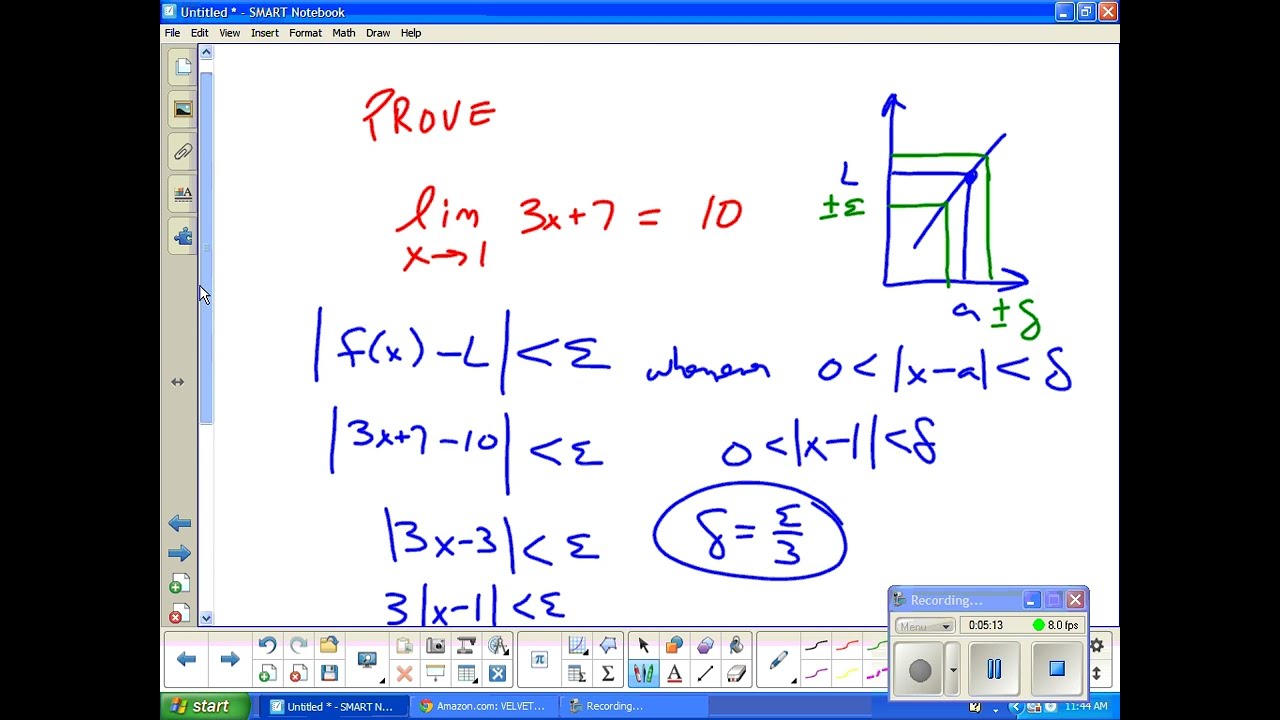This detailed image captures a screenshot of a virtual whiteboard presented in a landscape orientation, used as an interactive instructional tool. At the center of the screen, a digital notepad displays a mathematical problem along with step-by-step solutions. The predominantly handwritten text is rendered in red, blue, and some green, with the top section focusing on the word "PROVE" in red, and subsequent formulas and numerical notations mainly in blue. On the right side, various mathematical symbols and a small graph are present, including equations like "plus 8" and "plus 3." A backward '3' and a circled '3' can also be noted among the detailed annotations.

The left side of the screen features a vertical gray navigational pane, housing icons typically used for attachments and quick navigation, such as a paperclip and puzzle piece. Below these are blue navigational arrows. Alongside the pane is a blue elevator bar for scrolling. In the bottom right corner, a small tab marked "recording," along with numerical details, indicates that the lesson is being recorded, with a recording meter visible within this area. This illustrative, informational freeze-frame effectively doubles as a sophisticated virtual teaching aid, blending notational clarity with interactive elements aimed at a seamless educational experience.